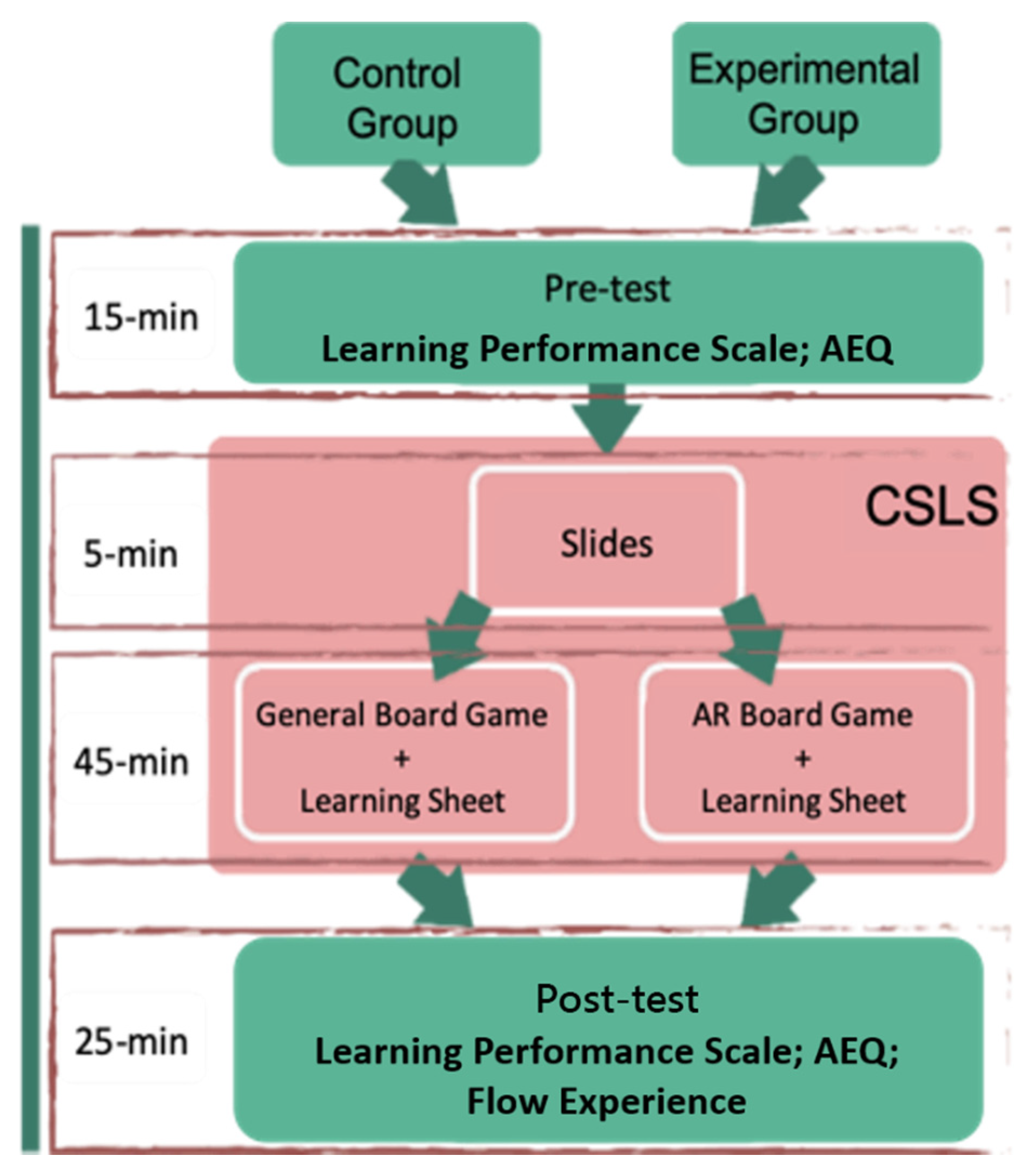This cross-sectional scientific drawing illustrates the detailed process of an experiment, comparing a control group and an experimental group. At the top, two green rectangular boxes labeled "Control Group" and "Experimental Group" initiate the flowchart. Both groups proceed similarly through the steps outlined below. The first step involves a green box labeled "15 minutes, Pre-test, Learning Performance Scale, AEQ," followed by a downward green arrow pointing to the next stage. This subsequent stage is a pink-red box labeled "5 minutes, Slides, CSLS." The flow then diverges into two options in separate pink-red boxes: either "45 minutes, General Board Game and Learning Sheet" for the control group or "45 minutes, AR Board Game and Learning Sheet" for the experimental group. The paths reconverge into a final green box labeled "25 minutes, Post-test, Learning Performance Scale, AEQ, Flow Experience." This organized chart visually details the experimental timeline and processes for both the control and experimental groups.